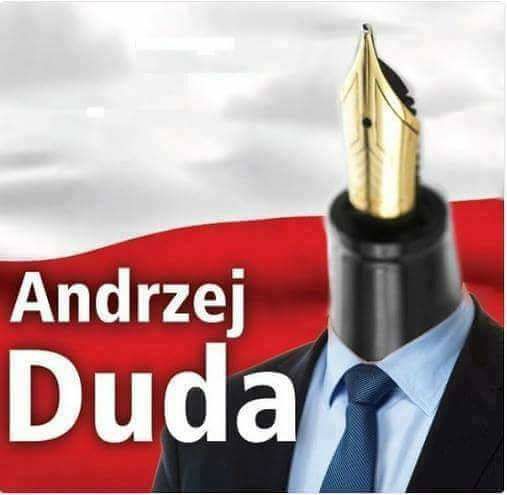The image depicts an intriguing visual composition resembling an advertisement or campaign graphic. Dominating the center is a headless black mannequin adorned with a sophisticated attire: a black suit coat, a light blue button-down shirt fastened fully to the collar, and a navy blue tie accented with small white polka dots. Replacing the mannequin's head is the gold nib of an old-fashioned fountain pen, adding an unusual yet striking element to the visual.

The text on the image spells out "Andrzej Duda" (A-N-D-R-Z-E-J-D-U-D-A) in a clean sans serif font, likely Calibri, spread over two lines. The first line reads "A-N-D-R-Z-E-J" in white font, while the second line features "D-U-D-A" in a slightly larger size. Positioned against the background, the top half of which displays a cloudy sky blending dark gray clouds with patches of white, and the bottom half exhibits a red section evocative of the flowing fabric of the Polish flag. Overall, the image skillfully merges elements of distinguished formality with creative artistry, emphasizing the name "Andrzej Duda" against the symbolic colors of Poland.